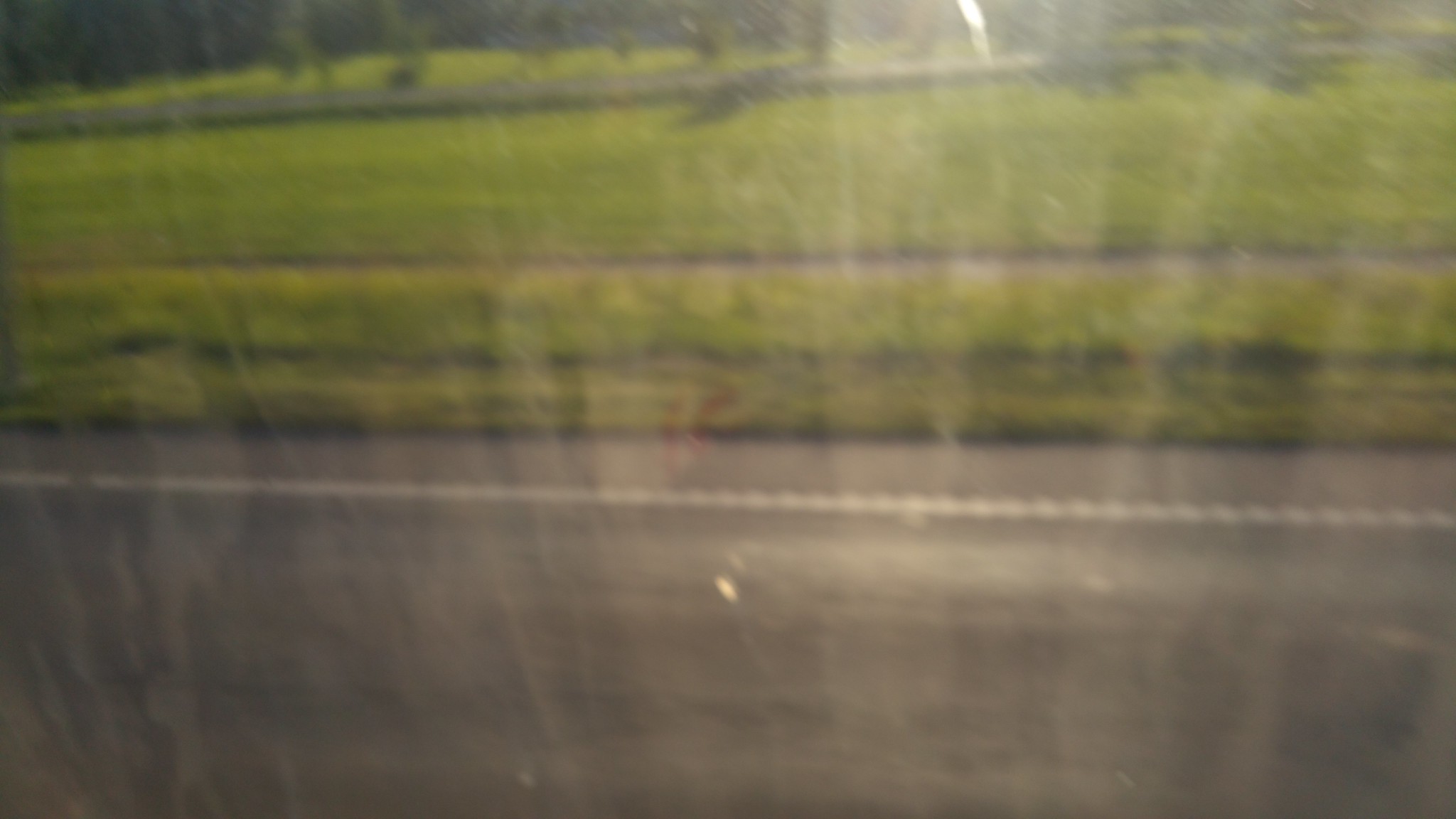This image appears to be taken from indoors, possibly through a window, as there is a subtle reflection visible on the glass. The scene captures a road stretching across the foreground, flanked by patches of grass. Adjacent to the road is a sidewalk. Beyond the first expanse of grass, there lies another area of greenery, suggesting an open field. In the distance, there is a gray structure, possibly another sidewalk or an additional road. The background is adorned with a cluster of trees, especially noticeable in the top left corner, where dense, dark foliage makes it difficult to discern further details. The overall view offers a tranquil, picturesque outdoor landscape as seen from the comfort of indoors.